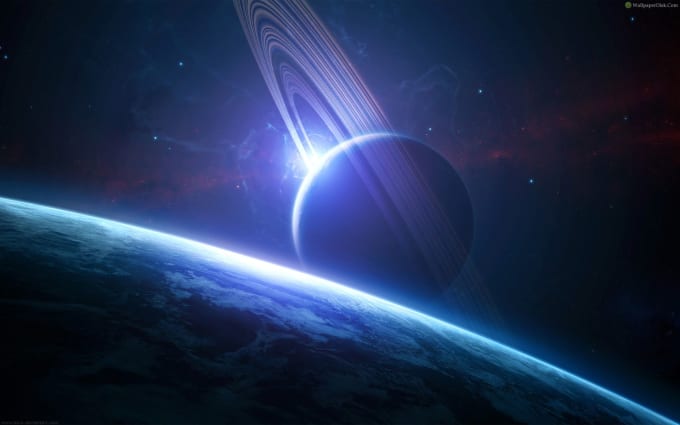This breathtaking digital artwork portrays an awe-inspiring space scape featuring a Saturn-like planet with prominent rings rising majestically above the horizon of a foreground planet, possibly Earth. The foreground planet, displayed in the lower left corner extending to the center of the left-edge, is characterized by dark hues interspersed with light-colored clouds, implying an atmosphere. Central to the image, the ringed planet's rings, depicted in shades of blue, white, purple, and a hint of orange, are tilted at an angle approximately 30 to 40 degrees, creating a dynamic and immersive perspective. The ringed planet itself appears dark, with a subtle illumination on its upper left side, contrasted against a distant dark sky populated with glimmering stars and a bright, white shining sun or star peeking behind its rings. Additional elements in the background include a reddish-purple nebula, adding depth and color to the dark, vast expanse of space. This masterful blend of colors and celestial details creates a striking and serene cosmic vista.